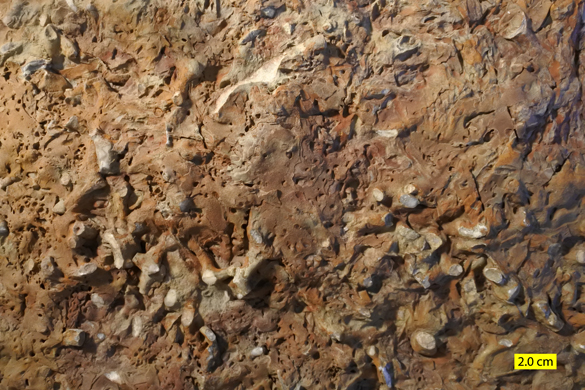This close-up photograph features an intricately detailed rock formation with varied textures and colors. The composition is dominated by earthy tones including browns, tans, grays, dark rusty reds, and light grays. In the bottom right corner, a yellow text box with black writing marks the scale as 2.0 cm, indicating a scientific context. The rocks display a striking mix of smooth, worn surfaces and porous sections, punctuated by occasional flat peaks. The overall appearance suggests a natural setting, potentially a cave wall or ground surface, capturing the complexity and variation within the minerals embedded in the scene.